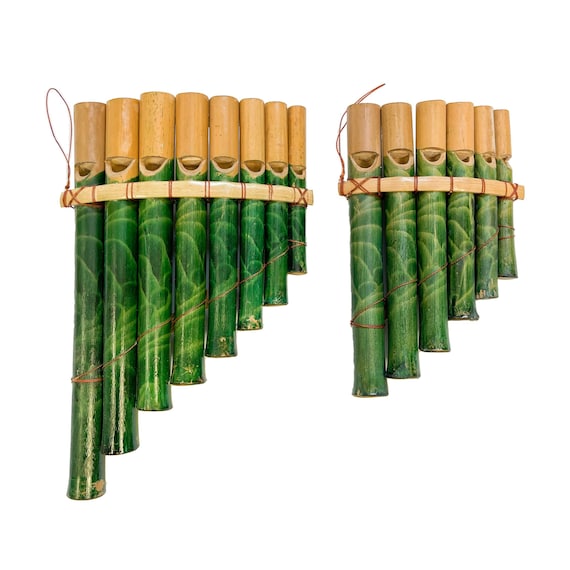The image showcases a display, possibly of items for sale, featuring intricately designed bamboo flutes. Each flute, set against a white background, is composed of varying numbers of green, hollow bamboo pipes arranged in descending order from the longest to the shortest. The pipes are painted a glossy green adorned with lighter green swirls. At the top of each pipe is a beige cap, which is the end blown into, and just below these caps are holes for airflow. 

One flute on the left contains eight pipes, while the one on the right has six. Both flutes have a horizontal strip of wood with vertical stripes, likely made from string, which helps secure the pipes together. This strip creates a step-like visual progression from bottom to top. At the end of each flute is a looped string, suggesting they can be hung as decorative pieces. Each flute's top end consists of natural bamboo color, contrasting with the green pipes, adding to the artistic and natural aesthetic of the instruments.